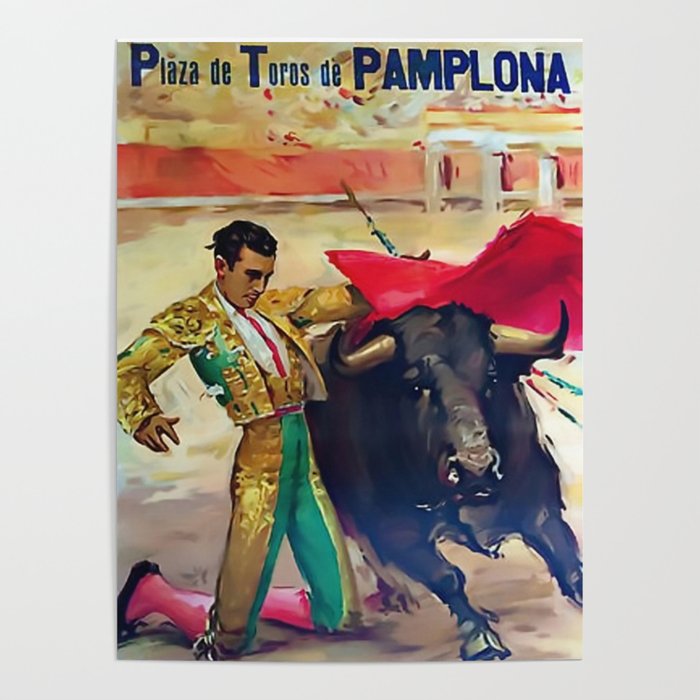The painted illustration depicts an elegant matador engaging in a dramatic bullfighting scene. He wears a striking outfit of green and gold, complemented by a red and white shirt, pinkish socks, and black shoes. The matador is skillfully maneuvering a vibrant red cape as he kneels in a dusty, light brown arena, his body almost touching the bull. The bull, appearing sorrowful, is captured mid-turn on the lower right side, with several swords already impaled in its back, highlighting the intensity and brutality of the spectacle. At the top of the image, bold blue text proclaims "Plaza de Toros de Pamplona," suggesting this could be a promotional poster for the renowned bullfighting events at this famous venue. The artwork, possibly created with watercolor, vividly brings the scene to life, capturing both the grace of the matador and the poignant struggle of the bull.